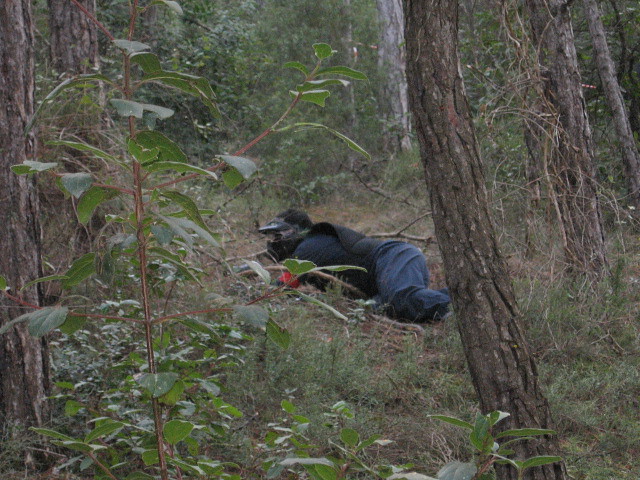In the midst of a dense forest scene during daylight, a man lies prone on the ground, partially concealed by underbrush and scattered pine trees. The lighting is subdued, suggesting an overcast day. The forest floor is a mix of grass, strawberry plants, and twigs, creating a rough, natural camouflage. The man is decked out in dark paintball gear, including a black helmet and vest, black shirt, and navy pants with knee pads. A red armband wraps around his left arm, contrasting sharply with his dark attire. His head is raised slightly, as if scanning the area for a target, and it appears he is gripping an obscured object behind a tree branch, possibly a marker. Tree trunks flank the scene, framing this tense and anticipatory moment in a paintball game.